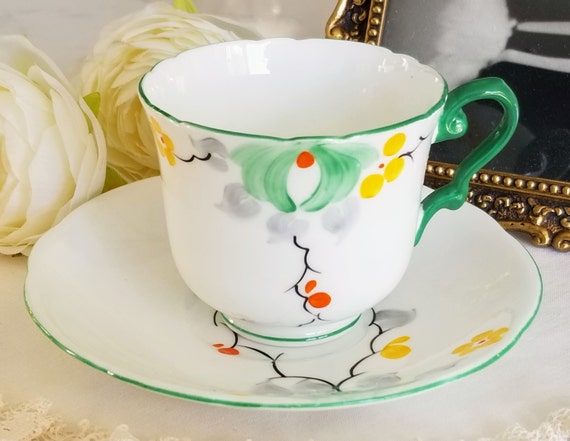The photograph captures a beautifully arranged white porcelain teacup and saucer set, accented with green details. The saucer, outlined by a thin green rim, features a delicate black floral design at its center. Surrounded by additional red and yellow dots with grey shading, this pattern adds an artistic touch. The matching teacup, adorned with a green handle and rim, showcases unique green banana-shaped motifs, red and yellow circles, and mild scalloping along the rim. Set against a white doily on a marble table, the background includes two elegant white peonies, adding a fresh natural element. To the right, an ornate golden-framed mirror with an intricate, almost ancient design, enhances the scene's overall sophistication and timeless charm.